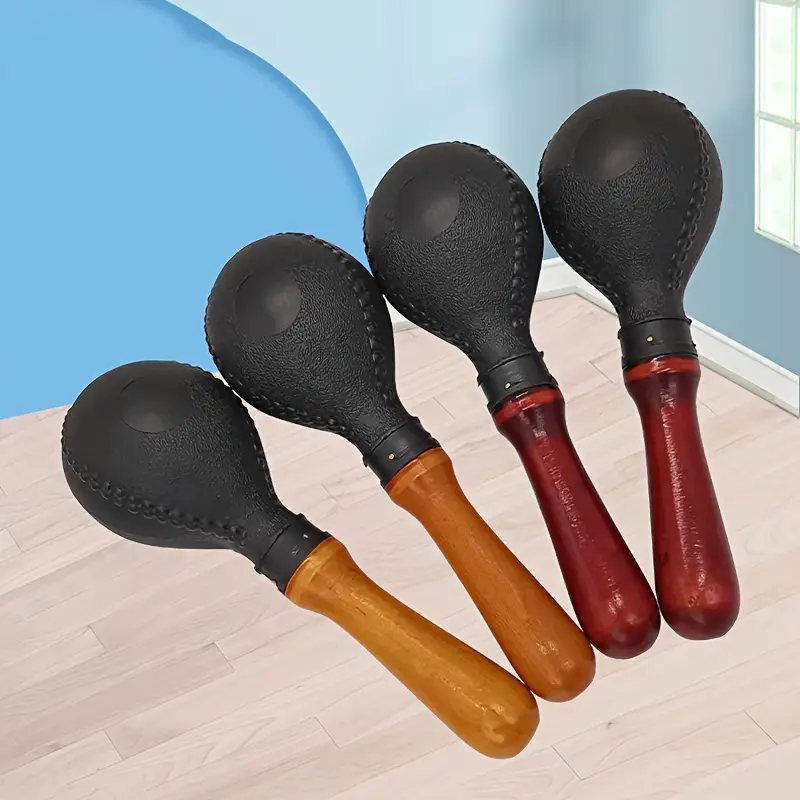The image depicts four juggler's clubs, suspended in midair against a light tan wooden floor. The clubs feature black leather heads and two distinct types of wooden handles: two clubs have light brown handles, while the other two sport rich burgundy-colored handles. The setting includes a blue-painted room with a partially visible window in the top right corner. The wall also displays an indistinct dark blue painting or mural. White trim accents the room, complementing the scene's aesthetic.